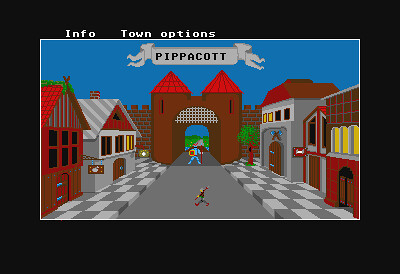The image appears to be a screenshot from a video game, depicting a digital, pixel-art style medieval town square. It is framed by a black border with a thin white line along the interior edge. At the top of the screen, white text reads "Info," "Town," and "Options." Below, in the center, a banner against a bright blue sky reads "PIPPACOTT" in uppercase letters, flanked by decorative swirls.

The town itself features a mix of brown and gray buildings, with a conspicuous castle gate situated centrally. The gate, constructed of brown material, boasts two small red-roofed towers. Emerging from the gate, a warrior clad in light blue and holding a gold shield stands on a gray road that cuts through the middle of the scene. A second, smaller character is depicted near the lower portion of the road.

The road is flanked by dark gray and light gray checkerboard sidewalks. On the left and right sides of the road, there are various buildings constructed in shades of red, white, and brown. A small tree is also located near the gate, adding a touch of greenery to the digital landscape. The entire setting evokes a quaint, medieval atmosphere typical of an artistic video game design.